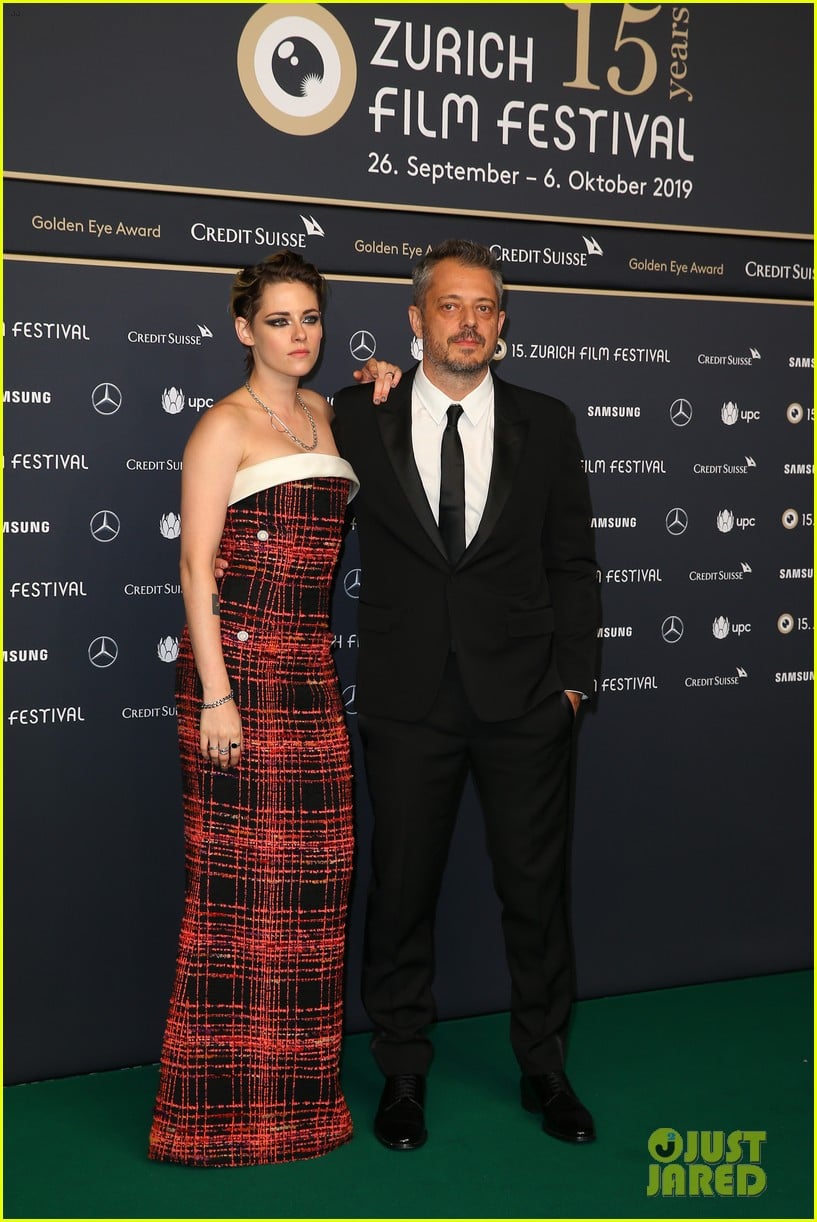This photograph captures a striking scene at the Zurich Film Festival, held from September 26 to October 6, 2019. The image features two people posing in front of a black backdrop adorned with logos of sponsors such as Credit Suisse, Samsung, UPC, and Mercedes-Benz, along with text celebrating "Zurich 15 Years the Film Festival." The backdrop, filled with tan and white font, serves as an elegant canvas for the subjects.

On the left stands a young woman, identified as actress Kristen Stewart. She wears a striking strapless red and black cross-hatched patterned dress, which features a white band of fabric across the top of the bust. Her accessories include a thin silver necklace, a bracelet, and several rings. Her dark hair is styled back, emphasizing her poised and elegant look.

Next to her is an older man dressed in a classic black suit with a white shirt and black tie. He sports short gray hair and a five o'clock shadow, adding a touch of rugged sophistication to his attire. The duo stands on a green carpet, which contrasts subtly with the formal ambiance of the event.

A watermark in the lower right corner indicates that the photo is credited to the celebrity tabloid magazine Just Jared. The photograph, vertically aligned, captures the full bodies of both individuals, effectively showcasing their stylish outfits and the glamorous atmosphere of the Zurich Film Festival.